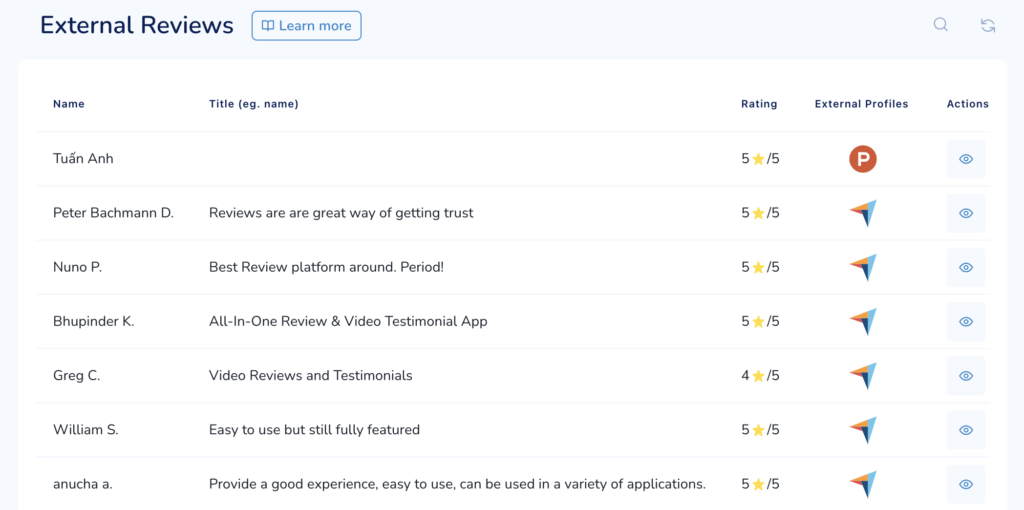The image displays a website interface featuring a sleek, light gray top bar. At the top, "External Reviews" is prominently written in black font. To the right of this text, there's a blue "Learn More" button inviting users to explore further. Below, labeled fields include "Name" and "Title" columns, each filled with various names and corresponding titles. The titles consist of phrases like "Reviews are a great way of building trust," "Best review platform around," "Video reviews and testimonials," "Easy to use but fully featured," "Provide a good experience," "Easy to use," and "Can be used in a variety of applications."

Each review holds a rating, most frequently receiving a five-star accolade, indicating high user satisfaction. Adjacent to the reviews is a column titled "External Profiles," displaying profile images. The topmost profile features a distinctive red circle with a white 'P' inside it, standing out against the other profile images.

To the far right, there's a category for actions, illustrated by a series of vertical blue boxes each containing a blue circle in the center. Finally, the website's header includes a light blue bar featuring a search icon on the left and two arrows forming a circular rotation symbol in the right corner, suggesting a refresh function.